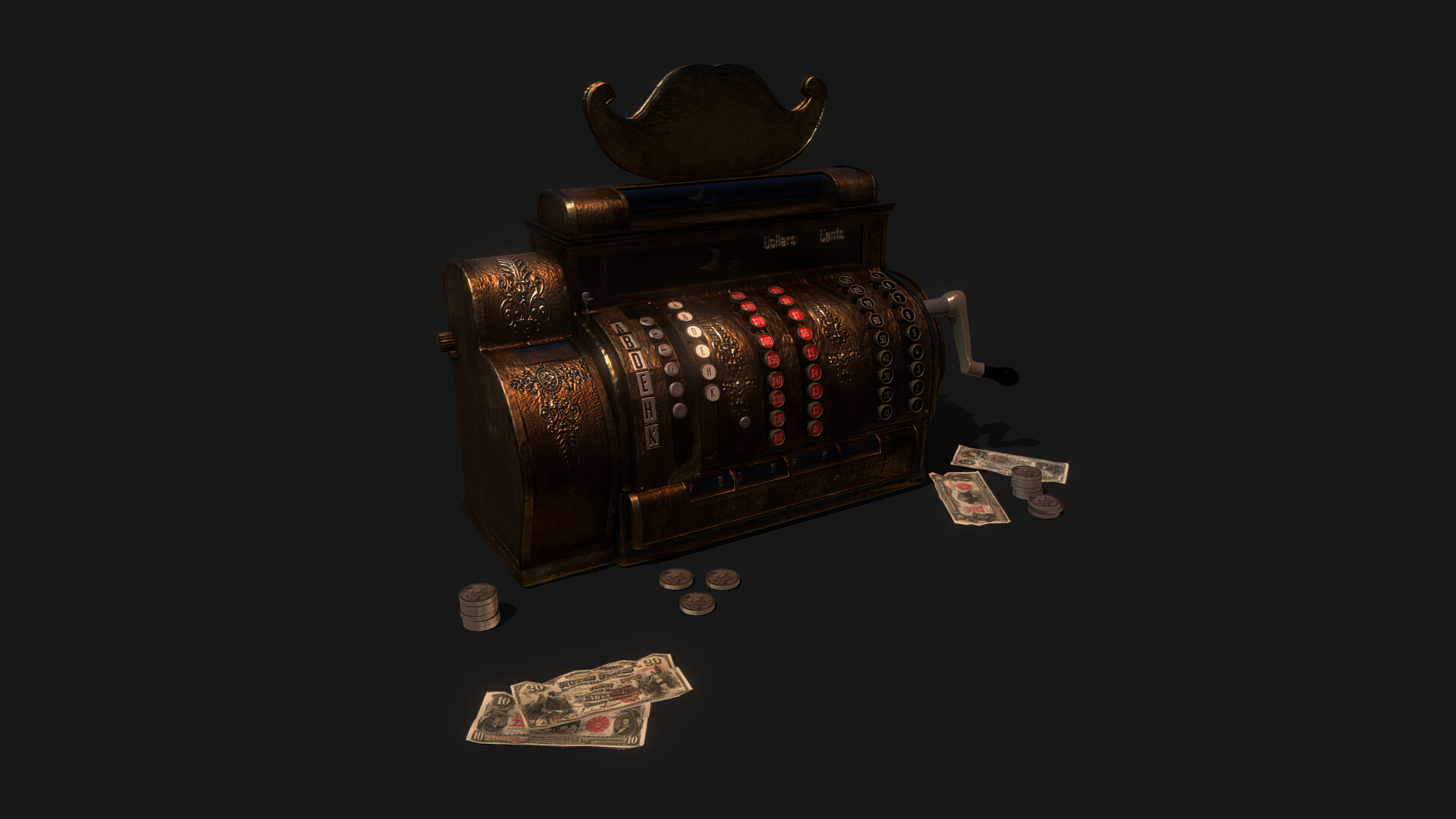The image depicts an ornately detailed, old-style cash register set against a solid, dark background. The cash register, rendered in a dark coppery-brown metal with intricate silver filigree and floral designs, features a variety of buttons and a silver hand crank on the right side. The left section shows keys labeled A, B, D, E, H, and K, while the front displays a mix of white, red, silver, and black buttons arranged in columns. In front of the register are four paper bills with red stamps, reminiscent of but not exactly like U.S. dollars, alongside several stacks of silver coins. The image, likely a piece of computer-generated art intended for a video game, manages to capture an almost photorealistic representation of an old-fashioned cash register amidst its gloomy backdrop.